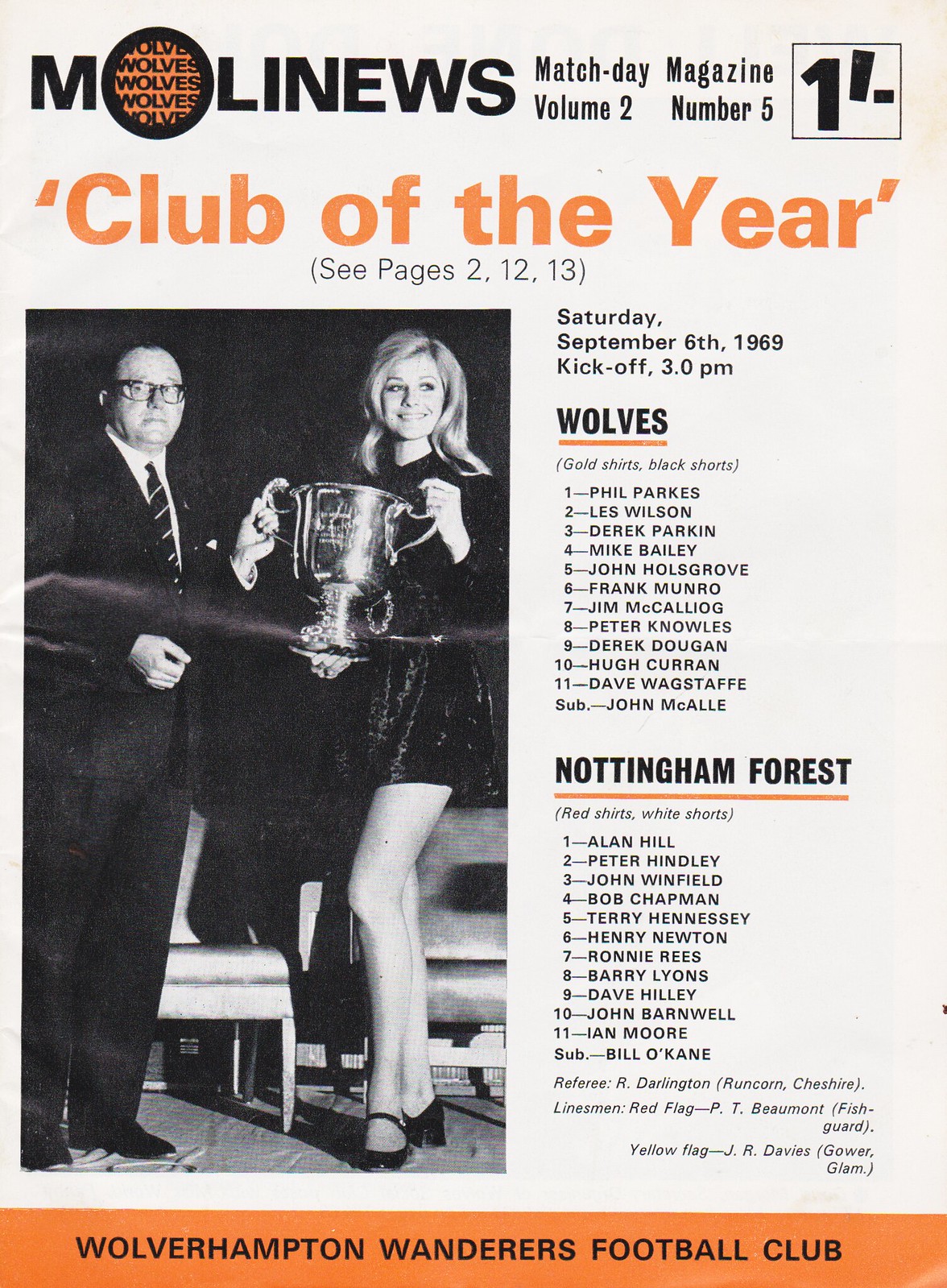The image depicts the front cover of a sporting event program for the Wolverhampton Wanderers Football Club, dated Saturday, September 6, 1969, with a kickoff time of 3 p.m. The program, titled "Moline News - Match Day," is Volume 2, Magazine No. 5. The top of the cover features an announcement for "Club of the Year," directing readers to pages 2, 12, and 13. Predominantly tan, black, orange, white, and various shades of gray color the cover.

On the left side of the image, a man in a suit and tie with glasses and a woman in a dress are holding a large cup-shaped trophy, symbolizing a significant achievement. The right side lists the rosters for the Wolverhampton Wanderers (Wolves) and Nottingham Forest. The Wolves' roster includes players such as Phil Parks (1), Les Wilson (2), Derek Parkin (3), and Derek Dugan (9), who are dressed in gold shirts and black shorts. Nottingham Forest's players, in red shirts and white shorts, include Alan Hill (1), Peter Hindley (2), John Winfield (3), and Dave Hilley (9). Additional text names the referee, R. Darlington from Runcorn, Cheshire, and the linesmen, P.T. Beaumont with a red flag and J.R. Davies with a yellow flag.

This program, detailed with specifics on the teams and match officials, would typically be handed out to attendees at the stadium entrance.